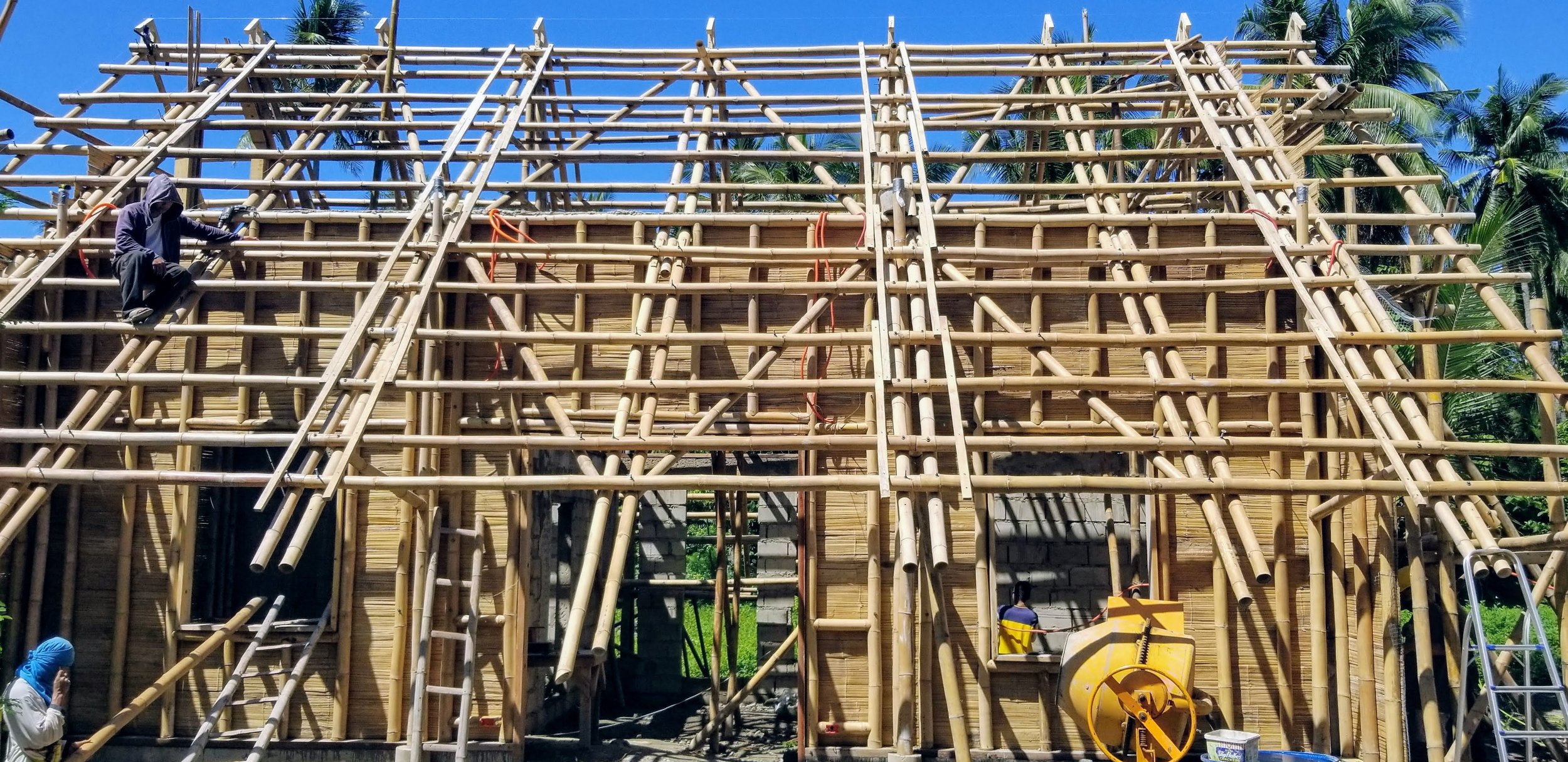This horizontal landscape photograph captures an active construction site of a light wooden house under a bright blue sky with palm trees in the background. The scene is bustling with activity, showcasing two individuals focused on their tasks. In the bottom left corner, a person wearing a blue hat is depicted holding a phone to their ear, while in the upper left corner, another person clad in a blue hoodie sits on the scaffolding. The wooden scaffolding, which might be made of bamboo, envelops the structure, reinforcing a predominantly wooden assembly. Various tools and equipment populate the foreground, including a ladder, a toolbox, and a yellow cement mixer on the bottom right. The construction site is marked by the prominent vertical and horizontal slats that form the framework for the roof, indicating that progress is well underway.